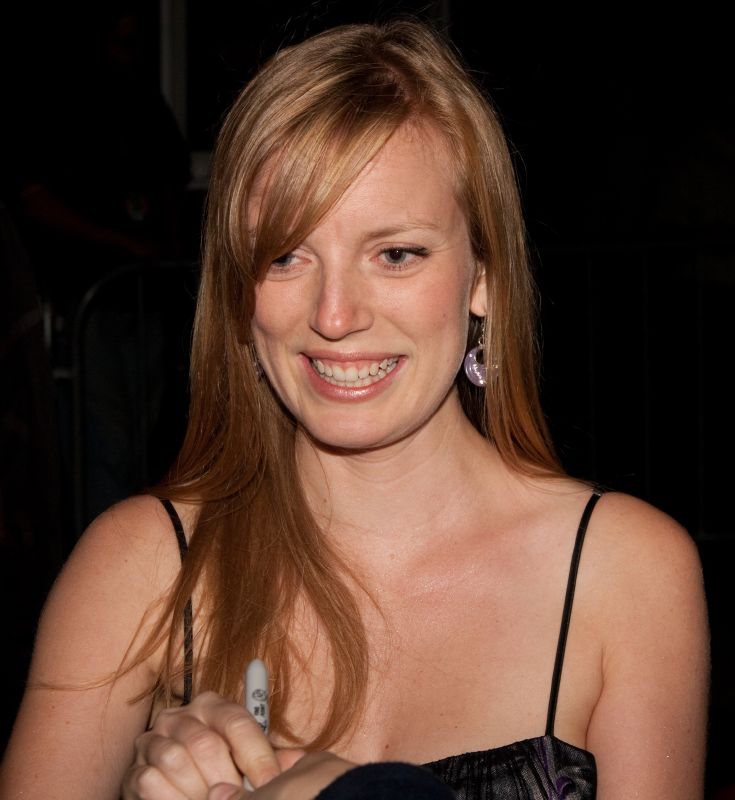The photograph is a striking portrait of a woman captured in a very close-up frame, visible from her upper chest to the top of her head. The background is a solid black, creating the impression that she is enveloped in a black void. She is wearing a thin-strapped black top, and her dangling crescent-shaped pearl earrings catch the light, adding an elegant touch to her look. Her long red hair falls by her chest, with a portion tucked behind her shoulder, revealing her left earring more prominently. Her face is adorned with minimal makeup, emphasizing her natural beauty, including a faint shine on her lips and visible freckles. Her green eyes are directed towards the lower left off-screen, and her mouth breaks into a broad smile, exposing both rows of her clean white teeth. Clutched in one of her hands is a gray Sharpie marker, positioned as if she is about to sign something or it is being handed to her by an unseen person whose hand just peeks into the frame from below. This detail, along with her poised and confident demeanor, suggests she might be a notable personality, possibly preparing to give an autograph.